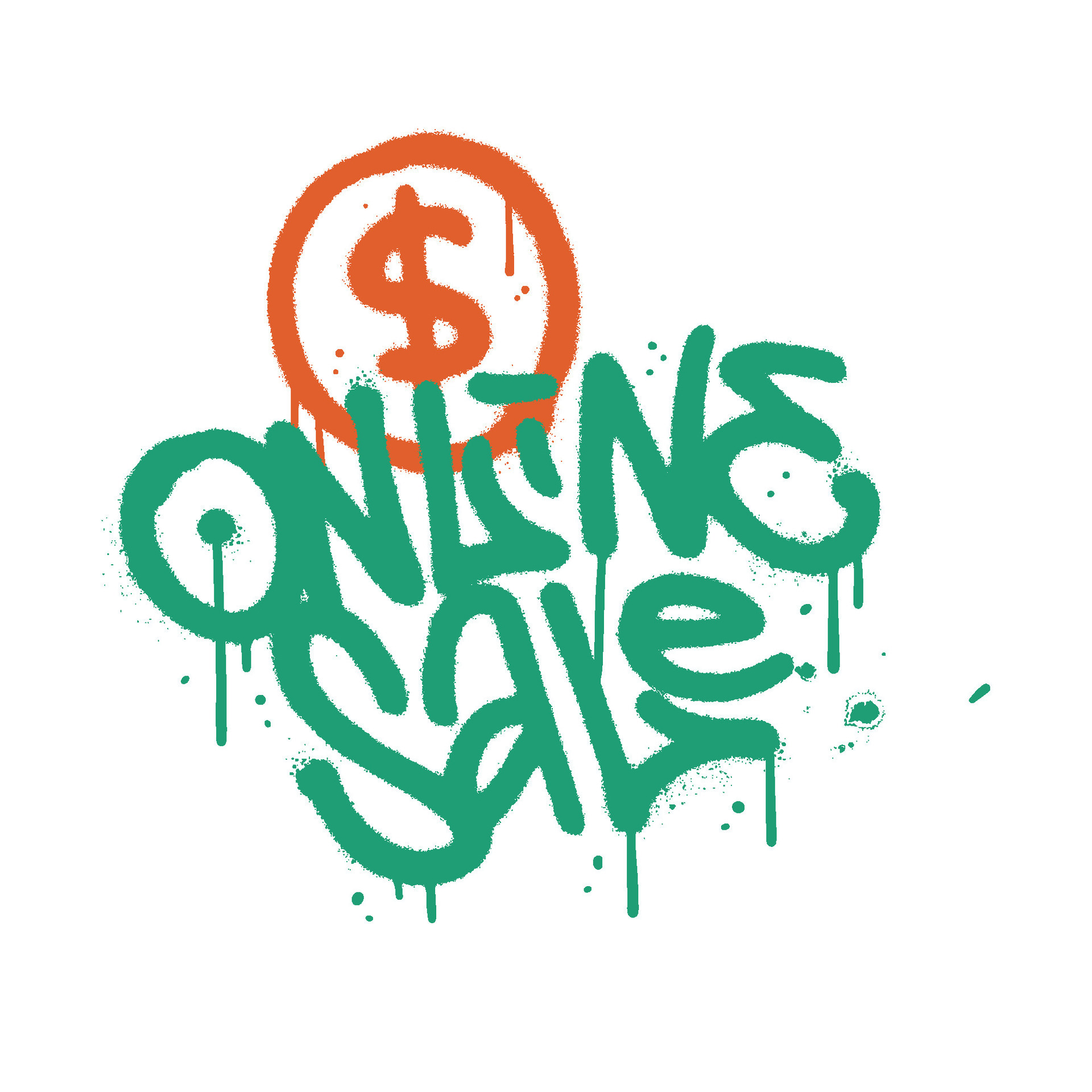The image features a minimalist, yet edgy design on a white background, reminiscent of street art or graffiti. Dominating the top is a thickly bordered orange circle, enclosing an orange dollar sign, both rendered with a dripping paint effect. Beneath this, in substantial green lettering also accented by dripping paint, the words "online sale" stand out. Splashes and drips of green and orange paint embellish the scene, enhancing the gritty, spray-painted aesthetic. The overall composition plays on the contrast of stark white against vibrant orange and green, mimicking the raw and unpolished style of urban street art.